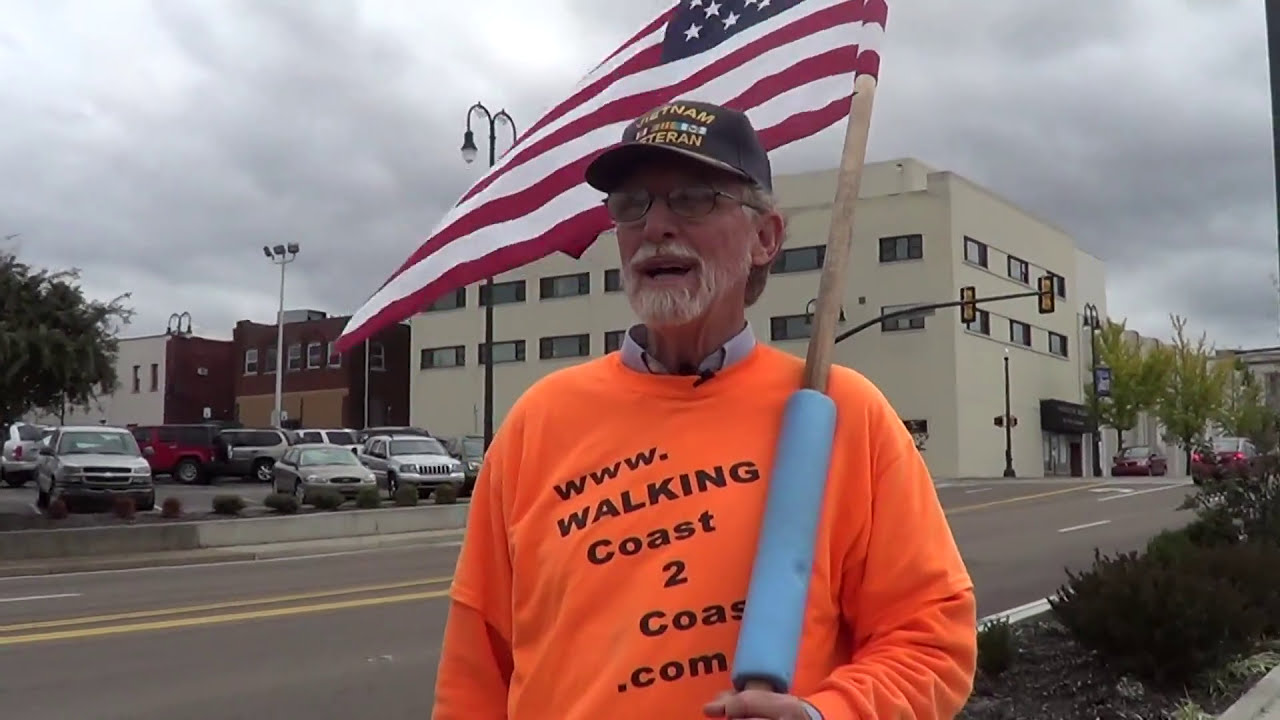In this outdoor landscape photograph taken on an overcast day, an elderly Caucasian man, donning gray hair and a white goatee, is captured walking along a sidewalk. He is dressed in a light blue collared shirt underneath a bright orange sweatshirt that prominently displays the text "www.walkingcoast2coast.com," serving as a walking advertisement for the website. He also wears a dark blue ball cap adorned with the words "Vietnam Veteran" in yellow, along with an array of military ribbons. The man holds an American flag on a short, wooden flagpole, which features a blue cushion wrapped around the pole for comfort as it leans against his shoulder.

The setting appears to be a small town's downtown area. In the background, you can see a white rectangular building, possibly commercial, which is accompanied by a parking lot containing about ten cars. A two-way street with minimal traffic runs adjacent to the sidewalk, with several cars visible. Additionally, there are trees and bushes adding greenery to the scene. The man appears to be walking on an island, surrounded by some brown dirt and bushes, positioned between the bustling street and the parking lot.